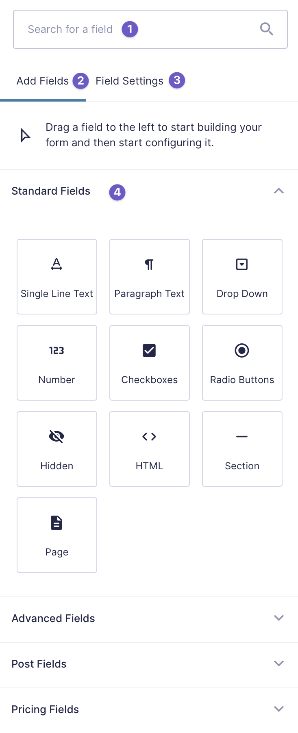This screenshot showcases a form-building interface with various elements highlighted using numbered, bluish-purple circles with white fonts. 

1. At the top, there is a search bar labeled with a circle numbered "1" in purple, meant for searching specific fields.

2. Immediately below the search bar, there is the "Add Fields" tab and the "Field Settings" tab. The "Add Fields" tab is selected, indicated by a horizontal aqua line beneath it and a circle labeled "2."

3. To the right of the "Add Fields" tab is the "Field Settings" tab, which is marked with a circle labeled "3."

4. Below these tabs, a prompt instructs users to drag a field to the left to start building their form and then to configure it. This section is followed by standard fields labeled with a circle numbered "4."

5. Under the "Standard Fields" header, there are several white boxes containing specific field options:
    - The first field is labeled "Single Line Text."
    - The second field is labeled "Paragraph Text."

Overall, the image provides a detailed visual guide for users on how to add and configure fields in the form-building interface.